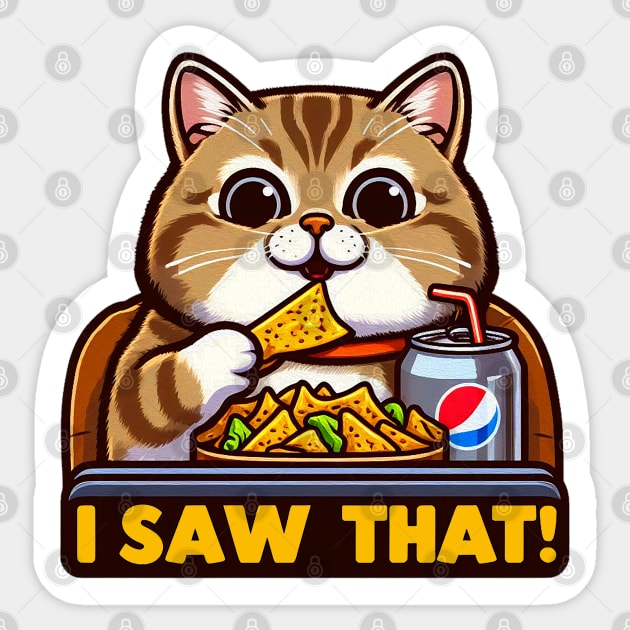This image showcases a detailed product photo of a sticker featuring a chubby orange-brown tabby cat with darker brown markings and white accents on its lips, chest, paw, and around its eyes. The cat, depicted in a cartoony style with pink ears, black stripes, and a smile, is sitting in a black or brown leather chair. In its paws, it holds a tortilla chip while staring directly at the viewer with a seemingly judgmental or knowing gaze. In front of the cat is a bowl of nachos with some green elements, and beside it is a silver Diet Pepsi can with a red bendy straw. The caption "I saw that" is prominently displayed at the bottom in yellow text on a black background. The entire sticker design is photoshopped onto a light gray backdrop with a padlock watermark running across it, hinting at its commercial nature.